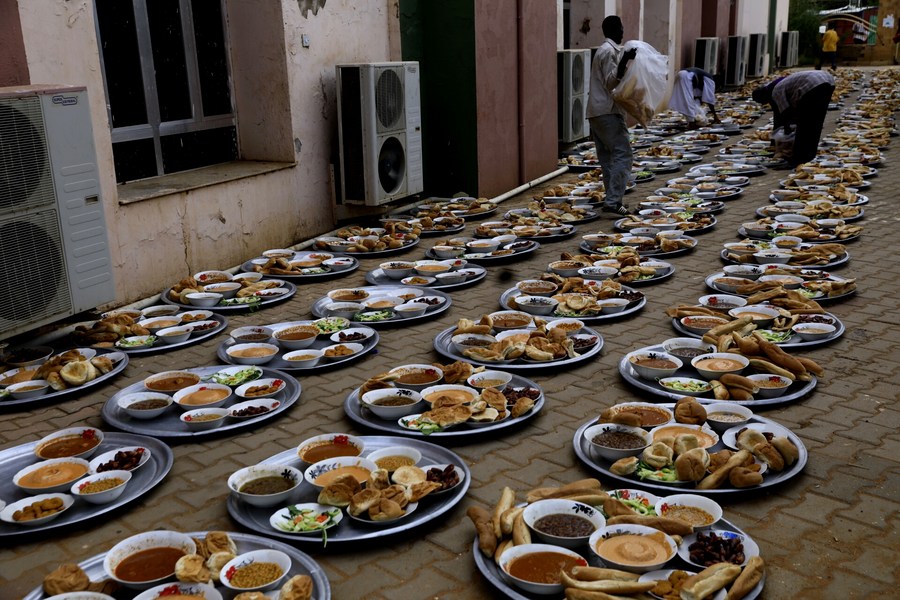The image depicts a densely-packed urban street likely in an African or possibly African-American community, showcasing a striking scene where hundreds of stone plates and large circular platters are meticulously arranged in long rows along the street. These platters, each holding an assortment of white bowls, contain various dipping sauces in red, black, and tan hues, a variety of soups, and loaves of bread. The background features older, run-down buildings with tan-colored walls, red columns, and side-mounted heaters. Multiple dark-skinned individuals are actively involved in placing food on the plates, creating an impression of a significant communal event. One man, dressed in clear plastic trash bags, is seen methodically distributing bread. The sheer volume of plates and the effort involved suggest an organized initiative, potentially aimed at feeding a large number of people, possibly as part of a charitable or community-driven activity.